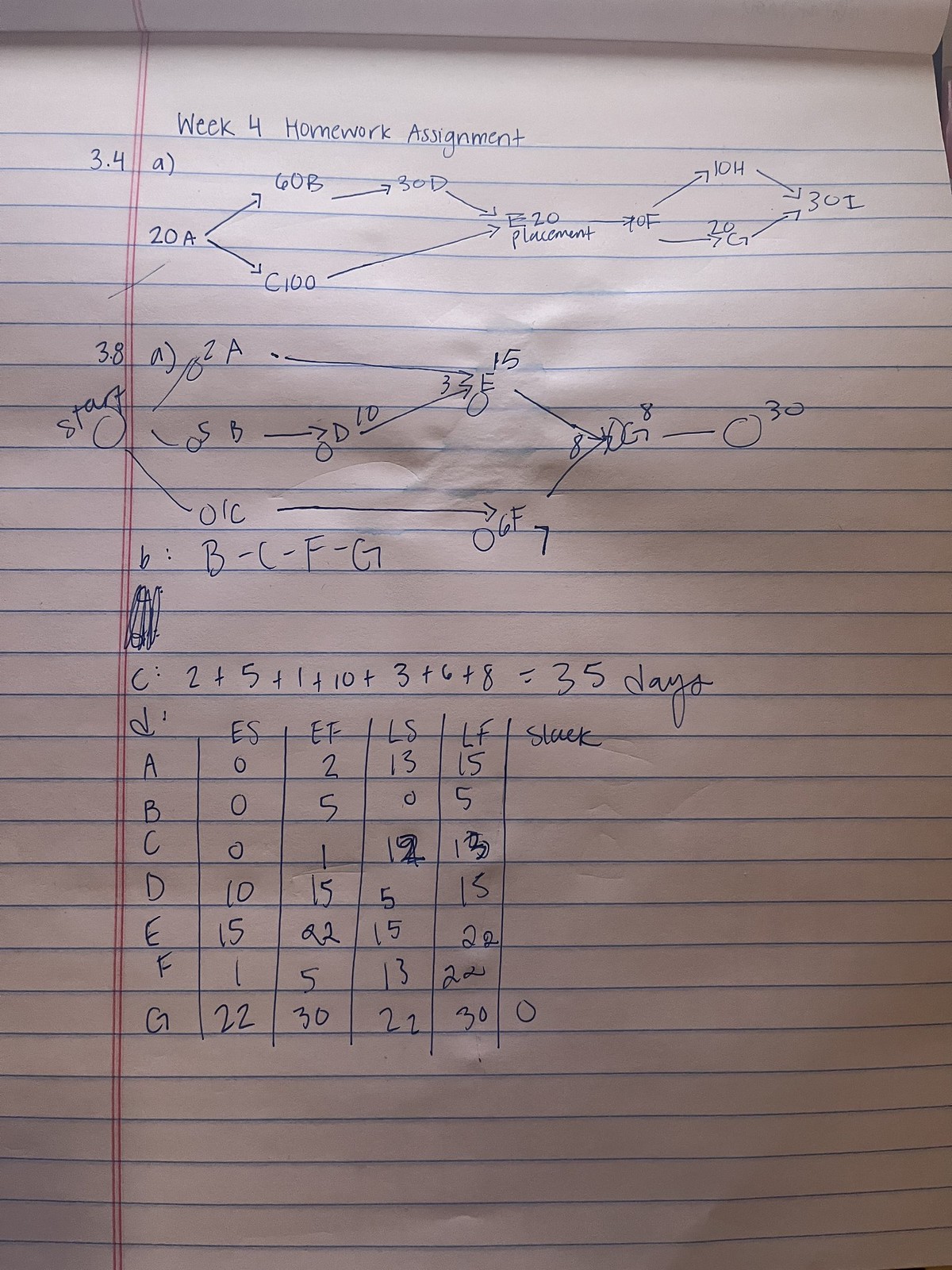A detailed caption for the given image:

"A close-up, color photograph in portrait orientation captures a slightly wrinkled white notebook page. The page features thin blue horizontal lines and a double thin red margin line on the left side. The top line of the page displays the heading 'Week 4 Homework Assignment' neatly written in blue ink. Beneath the heading, an array of numbers, letters, and arrows are scattered, indicating notes likely taken during a class. Prominently, there is an addition equation that reads, '2 + 5 + 1 + 10 + 3 + 6 + 8 = 35 days,' with the word 'days' elegantly written in cursive. Below the equation, a meticulously drawn chart spans 7 squares in length and 5 squares in width, filled with various letters and numbers. Shadows cast towards the right side add a subtle depth to the image, enhancing the visual texture of the slightly wrinkled paper."